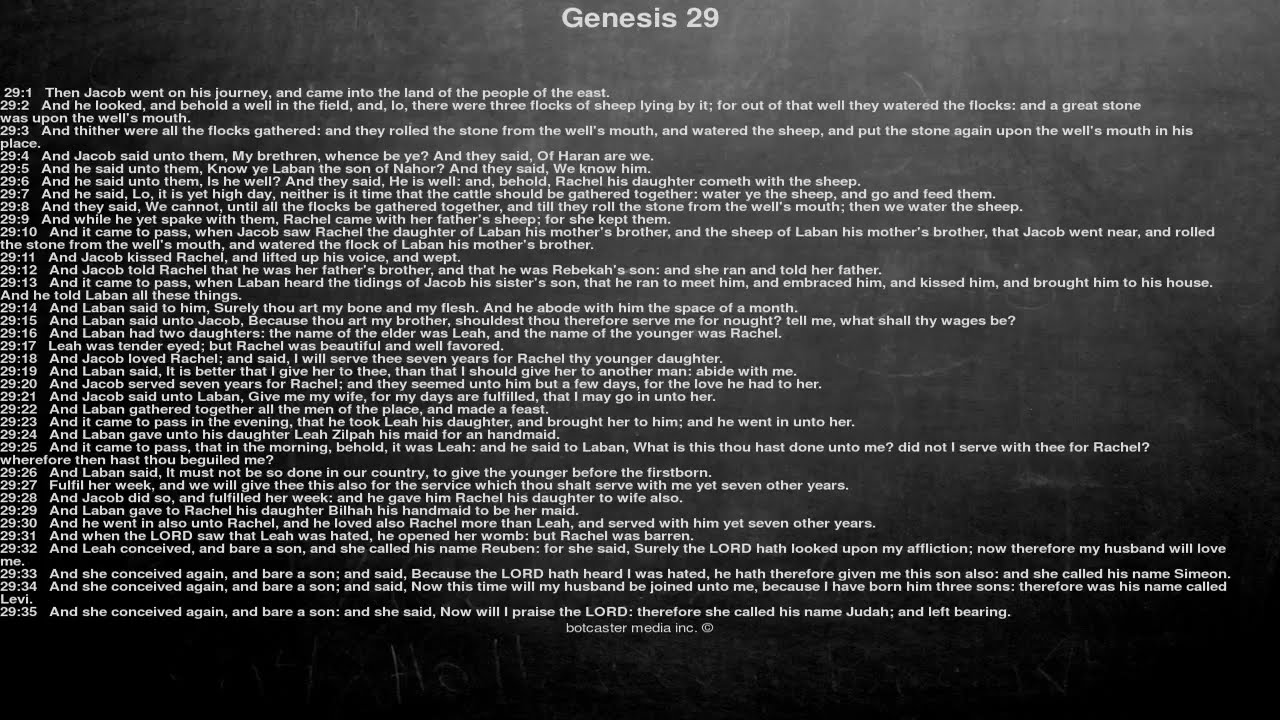The image displays a webpage from a Bible website, specifically featuring Genesis 29. The page consists entirely of Bible verses, starting from Genesis 29:1 and continuing to Genesis 29:35. The text is presented in small, white font against a black and gray background, making it somewhat difficult to read. The top of the page clearly titles the section with "Genesis 29." The verses begin with "Then Jacob went on his journey and came into the land of the people of the east," and continue describing Jacob's interactions and experiences, such as finding a well in a field. The document concludes with a copyright notice for Botcaster Media Inc.